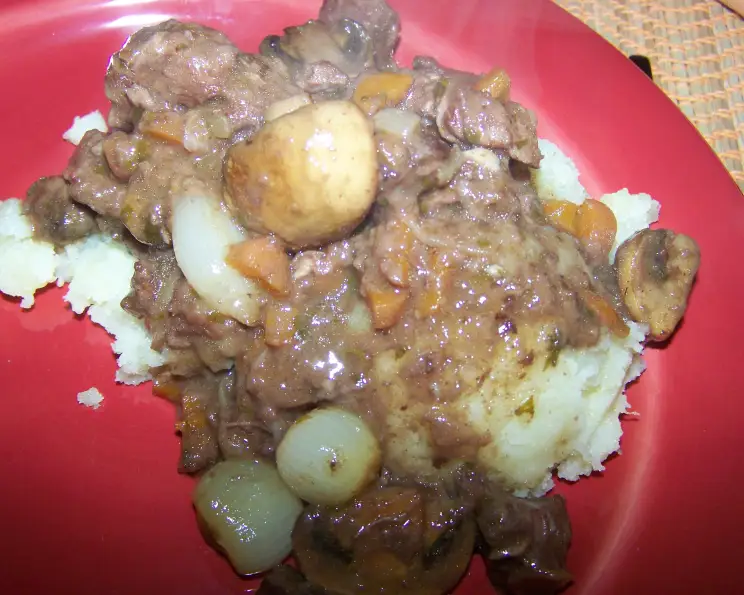A close-up image showcases a tantalizing prepared dish set atop a bamboo placemat with intricate string work and obscured black designs. The focal point is a red plastic plate holding a mixture of fluffy mashed potatoes smothered in glossy gravy. Scattered throughout the gravy are pieces of onions, mushrooms, and cut-up carrots, all enveloped in a rich sauce. The dish also features an unidentifiable type of meat, contributing to the hearty composition. The food arrangement under the bright light highlights its glistening texture and visible herbs sprinkled within the gravy, making the entire presentation visually appealing.